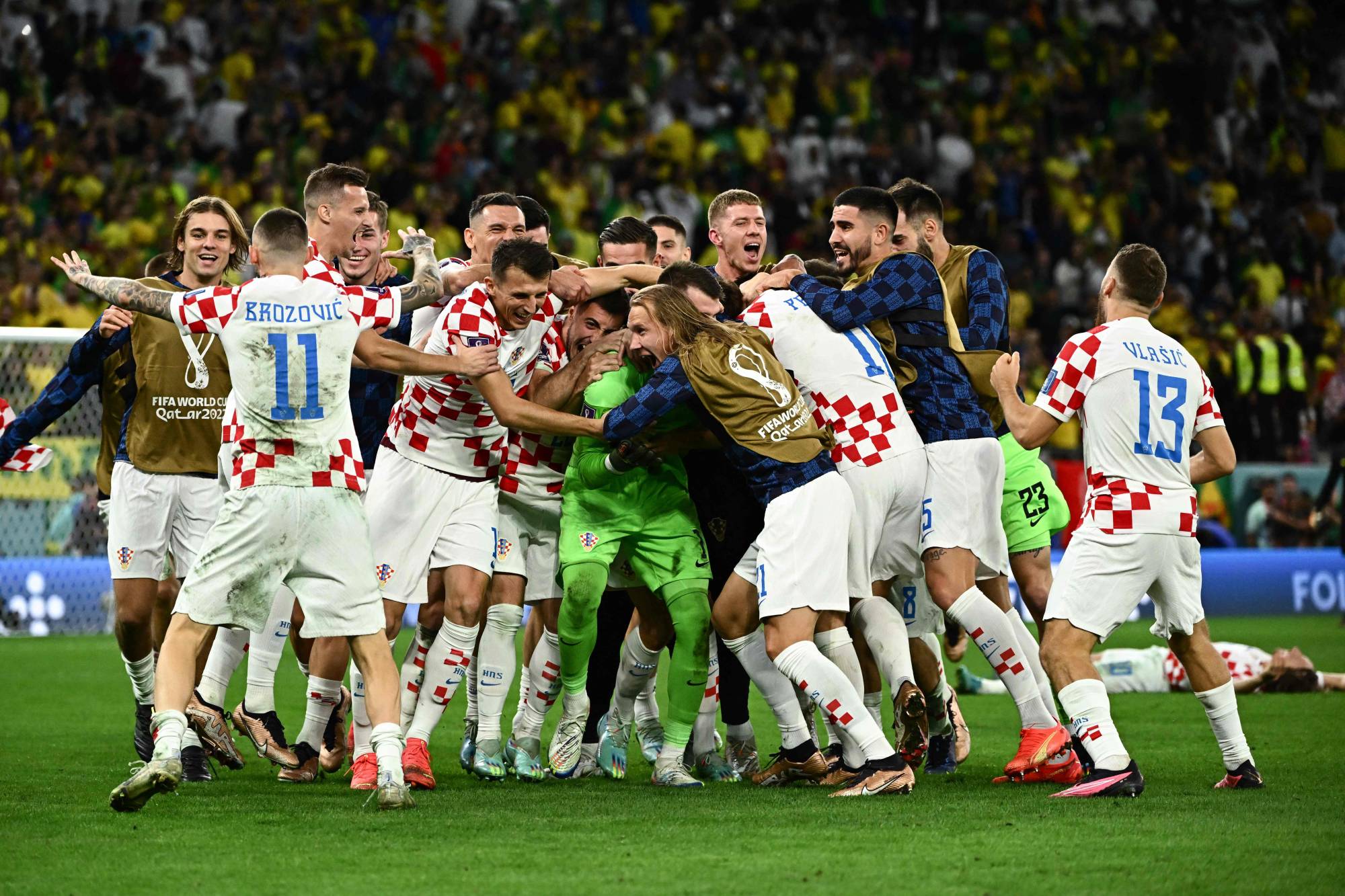The image depicts a joyous post-match celebration of a soccer team at the FIFA World Cup 2022. About 20 to 30 players form a large, animated huddle on the grassy field. The jubilant players, all young males, are embracing each other with outstretched arms, their faces glowing with happiness. 

The players wear a variety of uniforms: some sport white shirts with red and white checks, blue numbers, and names on the back, complemented by white shorts and socks. Others don navy blue and light blue checkered shirts paired with white shorts. Distinctively, a few players are clad in bright lime green shirts, shorts, and socks; they appear to include the goaltender, who is the focal point of the celebratory hug. In the background, a large crowd in the grandstand, muted but visibly filled with spectators primarily wearing yellow and white, adds to the festive atmosphere. Amidst the huddle, one player lies exhausted on the ground, encapsulating the intensity and elation of the moment. The scene is a vivid display of triumph and camaraderie on the vibrant green turf.